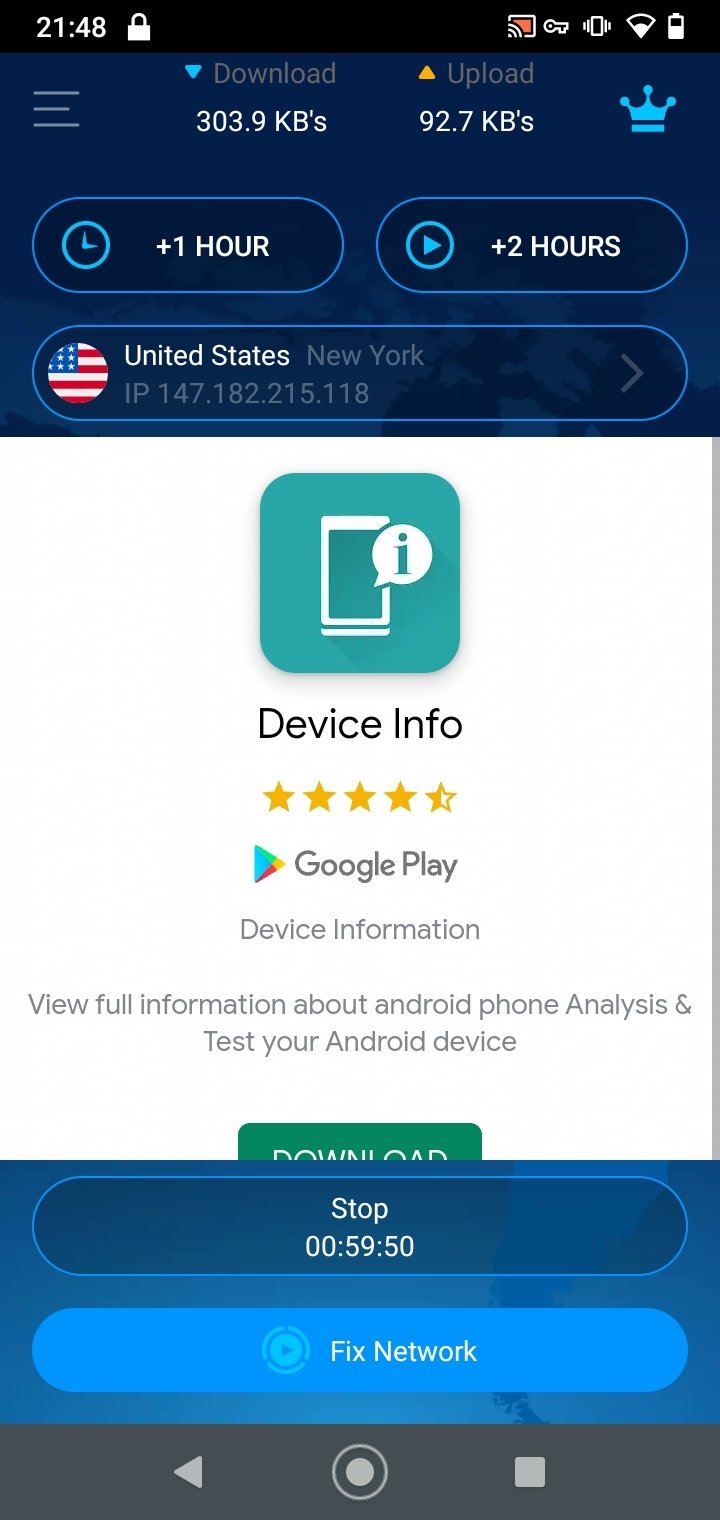**Detailed Screenshot Description:**

The screenshot appears to be taken on a smartphone, with the time displayed in the top left corner reading 21:48. Adjacent to the time is a lock symbol, indicating the device is locked. In the top right corner, several status icons are visible, including Wi-Fi connectivity, battery level, and additional symbols which are not clearly discernible.

The upper part of the screen features a blue background with a few notable elements. On the far left is a menu icon, and next to it is a "Download" label with the text "303.9 KBs" underneath, indicating the current download speed. Following this, there is an "Upload" label, accompanied by the text "92.7 KBs," signifying the upload speed. Towards the upper right, there is a crown symbol.

Beneath these elements are two prominent buttons: the button on the left is labeled "+1 Hour," and the button on the right is labeled "+2 Hours." Below these, there is another button labeled "United States, New York, IP 147.182.215.1118".

Continuing downward, there is a white box featuring a mobile device icon set against a light blue background, with the label "Device Info" under it. Following this, there is a rating of four and a half stars, and a description that reads: "Google Play device information, beautiful information about Android phone analysis, and test your Android device". Adjacent to this description is a green "Download" button.

The blue background extends to the bottom part of the screen, where there is a button labeled "Stop" with a timer showing "5950". Additionally, there is a brighter blue button labeled "Fix Network".